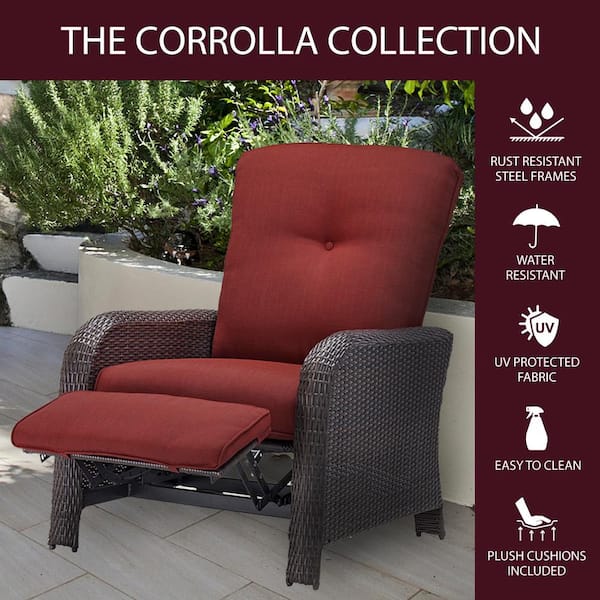Here we have an advertisement featuring an elegant outdoor patio chair from the Corolla Collection. The image showcases the chair in a high-end patio area that is tastefully tiled with light beige and white tiles, set against a backdrop of greenery and flowers neatly arranged in planters along a retaining wall. The chair itself is crafted from dark brown, rattan-like wicker and is complemented by plush, cinnamon-colored cushions. It includes a reclining footrest also upholstered in the same cinnamon fabric. 

At the top of the image, there's a maroon border with "Corolla Collection" written in white. The right side of the image lists the chair’s notable features, each accompanied by relevant icons: rust-resistant steel frames (depicted by water droplets), water resistance (indicated by an umbrella icon), UV-protected fabric (shown with a UV shield), easy-to-clean material (represented by a spray bottle), and plush cushions included (illustrated by a hand pressing on a cushion with arrows highlighting the softness).

This detailed setting and comprehensive description highlight the chair's comfort and durability, making it a stylish yet practical addition to any outdoor space.